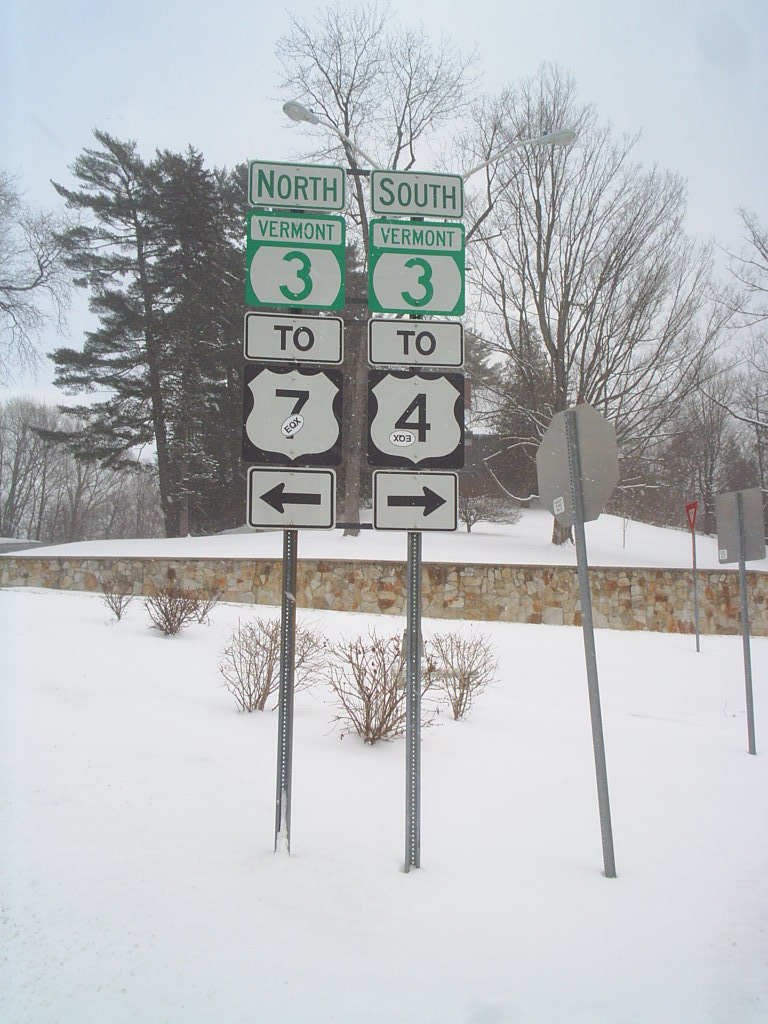A snowy outdoor scene featuring multiple road signs. The foreground prominently displays two identical stacks of street signs, with the left indicating "North Vermont 3 to 7" and the right indicating "South Vermont 3 to 4." Each of these signs has a directional arrow, with the left pointing left and the right pointing right. To the right of these signs are a stop sign and another square-shaped sign, both facing away from the camera. The ground is blanketed in a thick layer of snow, with scattered small bare shrubs and larger trees dotting a snow-covered hill in the background. A low, gray-and-tan stone wall, partially covered in snow, stretches horizontally across the mid-ground, delineating the hilly backdrop. The entire scene is framed by a white, overcast sky, giving it a distinctly wintery atmosphere.